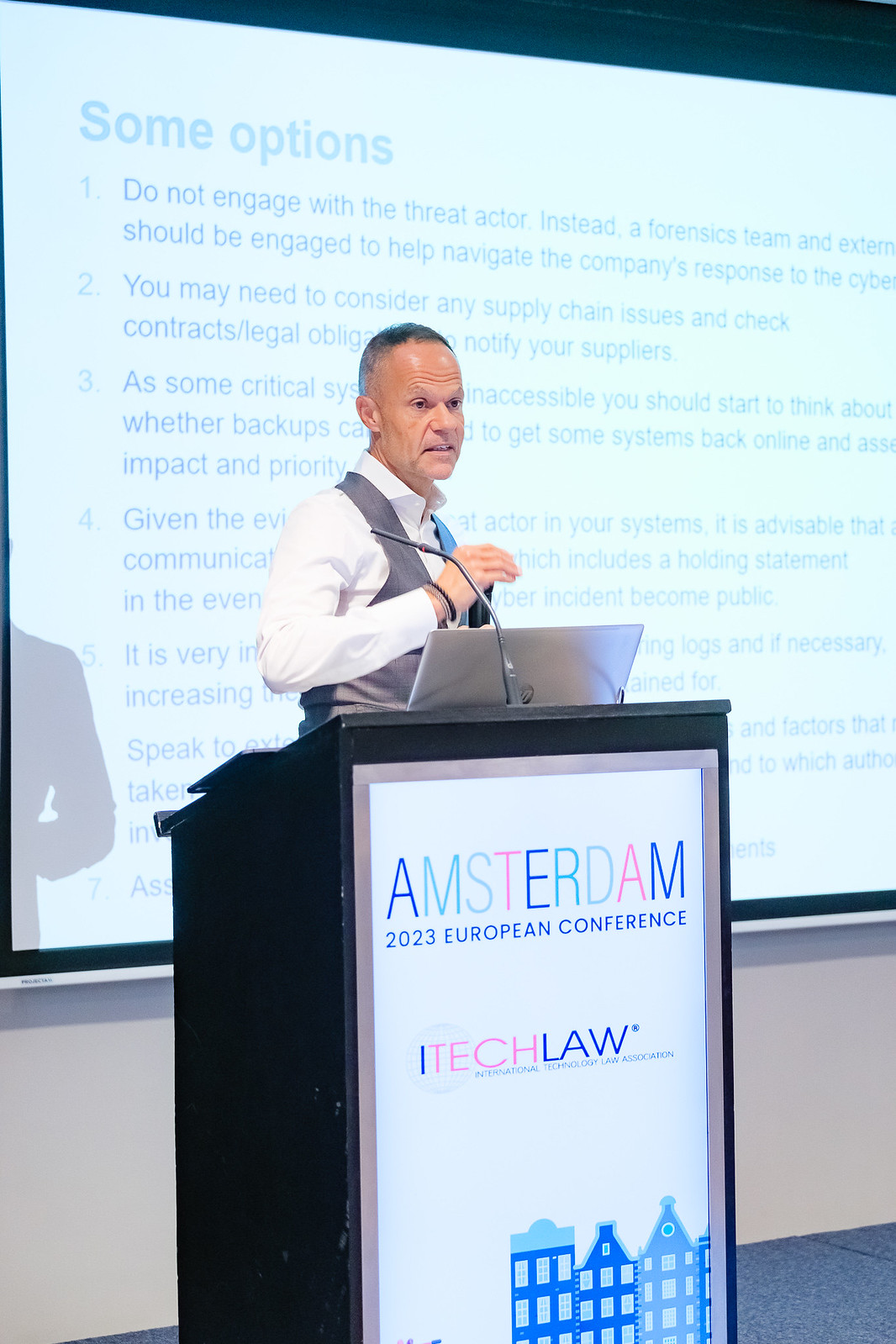In this detailed image, a man with short gray hair and fair skin is giving a presentation at the Amsterdam 2023 European Conference on I-Tech Law. Dressed in a white button-down shirt with an open collar and a gray vest, he stands behind a black podium adorned with vibrant multicolored text on a white background that reads "Amsterdam 2023 European Conference" and prominently features "I-Tech Law". His computer, a silver laptop, rests open on the podium, allowing him to navigate his PowerPoint slides projected behind him. The projection displays light blue text on a white background, including a numbered list. The backdrop also includes an illustration of Dutch-style row houses. A very thin microphone is clipped to him, ensuring clear audio delivery. The room is softly lit, with blue carpeting and white walls. The man's shadow is faintly visible against the left edge of the projection, adding depth to the scene.